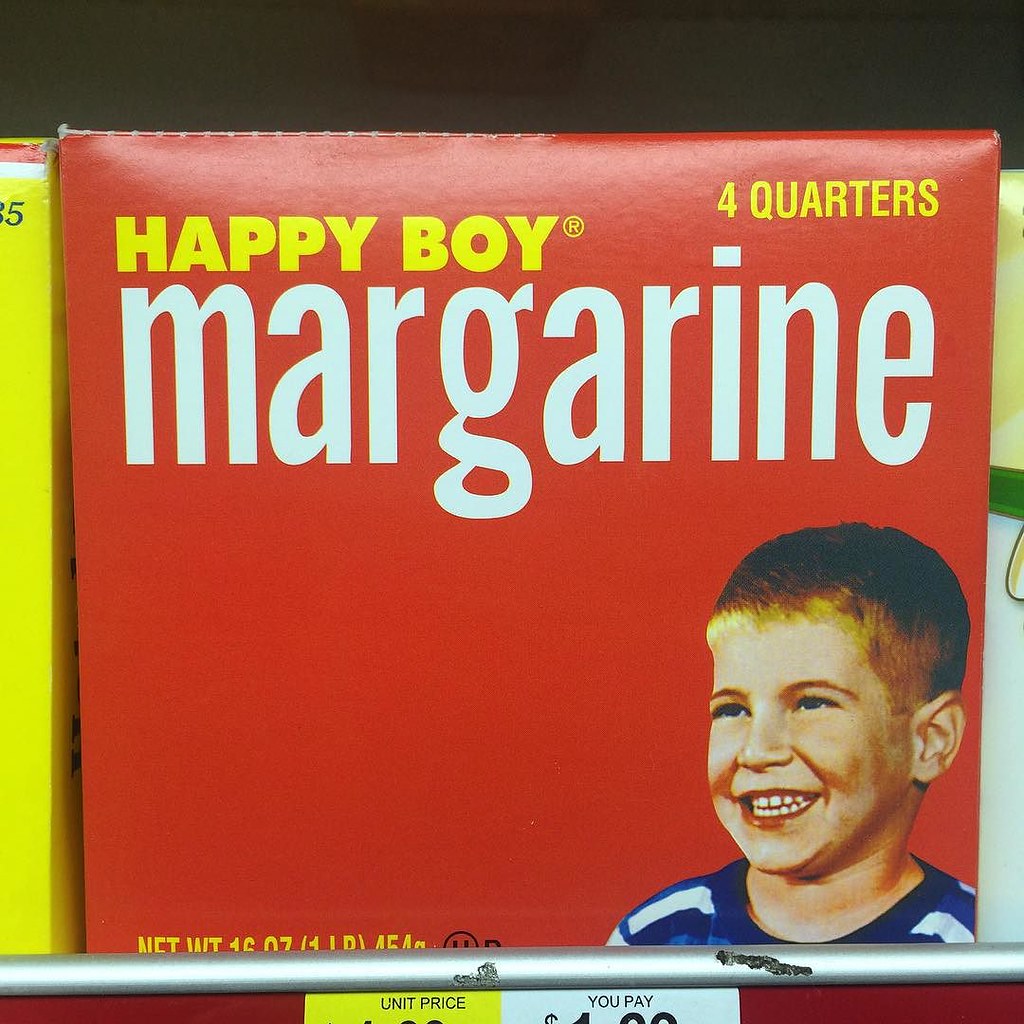The image captures a shelf in a marketplace, prominently featuring a product in a red box that dominates the frame. In the background, there are glimpses of shelf space and parts of adjacent products. The red box is the focal point, with vibrant yellow font in the upper right-hand corner proclaiming "Four Quarters." Just beneath this, also in yellow font, is the brand name "Happy Boy," marked with a registered trademark symbol. The largest text on the box, written in bold white font, reads "Margarine," making it clear what the product is. In the bottom right-hand corner of the box, there's a cheerful illustration of a young boy's face, smiling and dressed in a blue and white striped shirt. The box also indicates that the net weight of the margarine is 16 ounces.